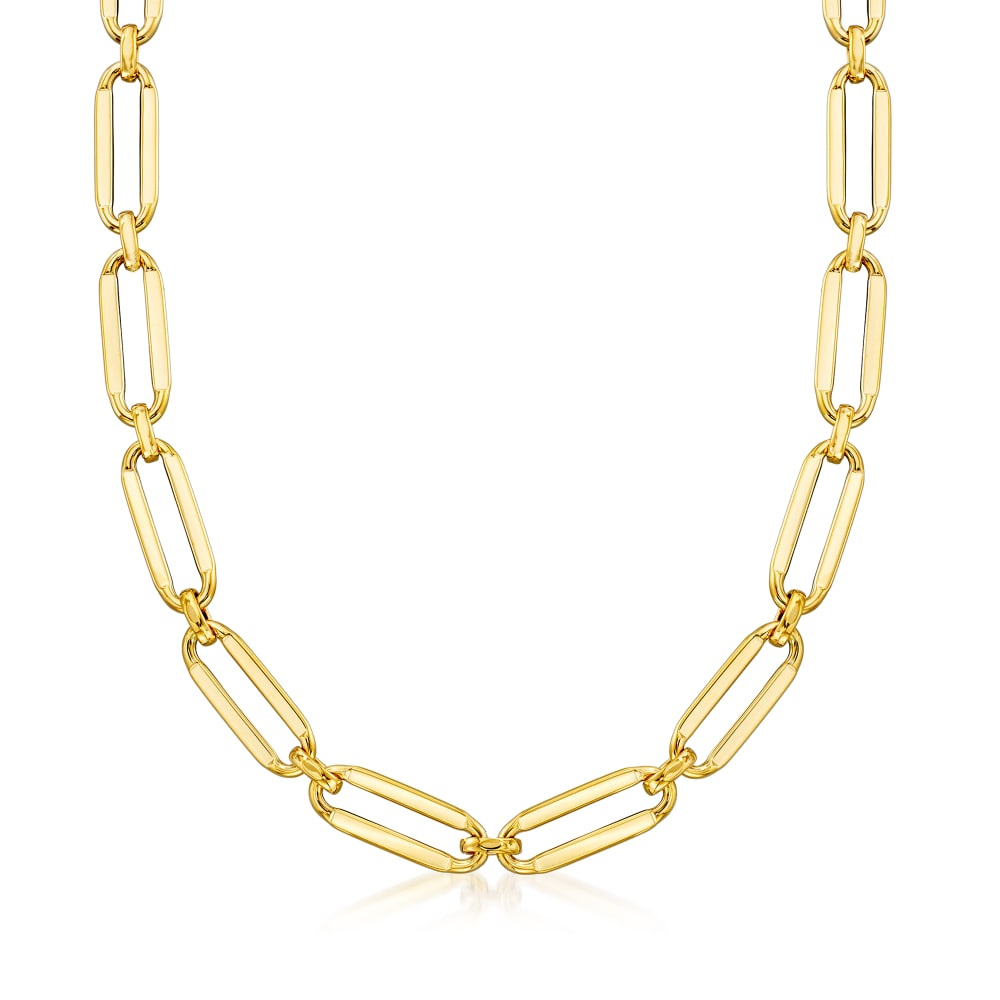The image is a close-up photograph of a gold necklace set against a white, almost non-existent background, resembling a stock image. The necklace forms a U-shape, starting from the upper left and right corners of the image and connecting at the bottom middle. It consists of twelve elongated, oval-shaped gold links with round ends, which are connected by smaller, circular gold rings. The gold links appear shiny with varying color tones, featuring a slightly different hue in the middle compared to the edges, which are shinier. Some portions of the links have a light pinkish reflection due to their shine. At the very bottom of the image, there's a subtle light gray reflection of one of the small gold rings and parts of the connected links, giving the gold a somewhat transparent, glass-like appearance.